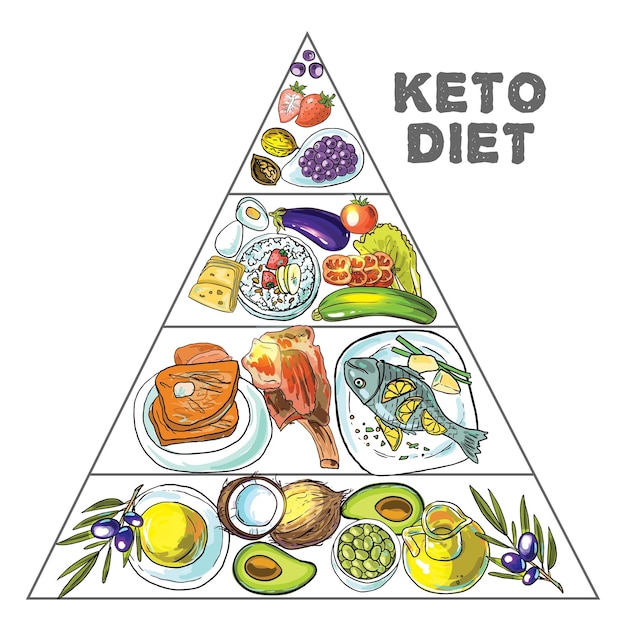This image illustrates an animated, cartoonish food pyramid set against a stark white background. In bold dark gray text at the upper right corner, it reads "Keto Diet," indicating it is a dietary guide. The pyramid is divided into four sections. The topmost, smallest section features an assortment of fruits and nuts: strawberries, purple grapes, blueberries, and a walnut. Below it, the next section showcases zucchini, tomatoes, lettuce, eggplant, a bowl of oatmeal, and cheese. The third section from the top includes various meats: a whole fish garnished with lemon, ham, a turkey leg, and possibly salmon steaks. The largest, bottom section displays a rich array of healthy fats: avocados, a coconut, olives with branches, a carafe of oil, a bowl of oil, and a tea glass. Each element is depicted in a lively, animated style, emphasizing the keto diet structure through detailed illustrations.